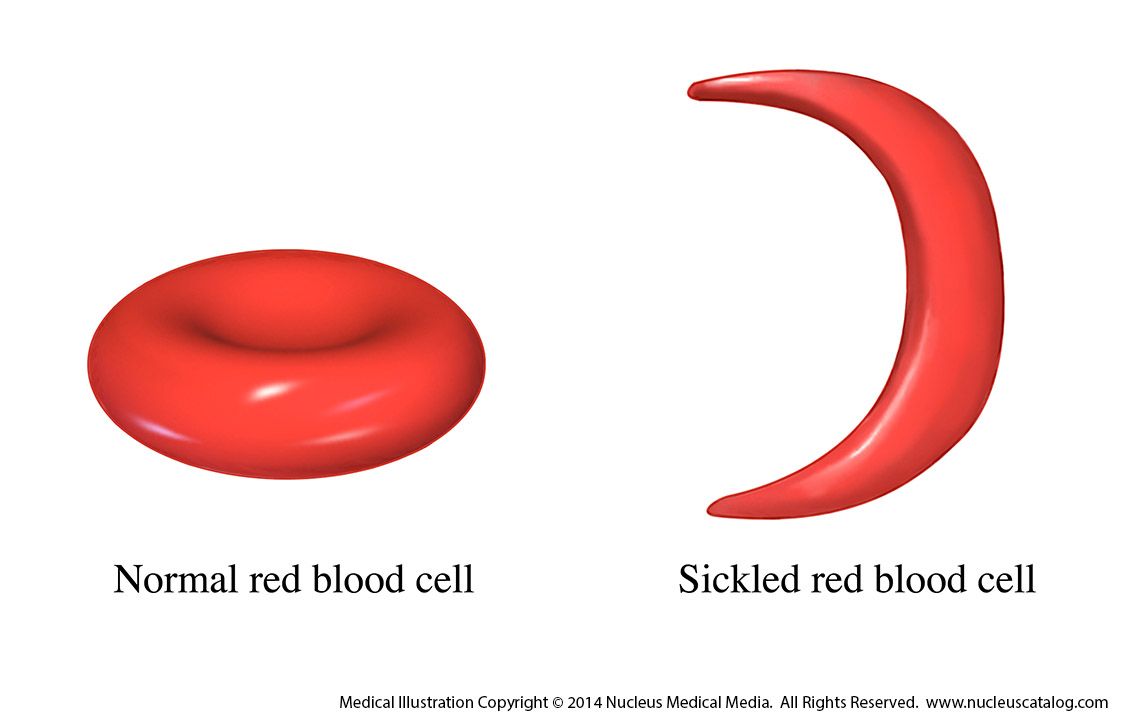The medical illustration depicts two types of blood cells against a white background, emphasizing their distinct shapes and conditions. On the left, there is a large, circular red blood cell with a central indentation, resembling a donut. This cell has white highlights on its surface, indicating reflected light and is labeled "normal red blood cell" in black text beneath it. To the right, a red crescent-shaped blood cell is shown, also with light reflections on its edges, and is labeled "sickled red blood cell" in black text. The bottom center of the image features the disclaimer "medical illustration © 2014 Nucleus Medical Media. All rights reserved. www.nucleuscatalog.com" in small black print. This illustration effectively contrasts the appearance of a healthy red blood cell with that of a sickle cell, offering a clear visual comparison for educational purposes.